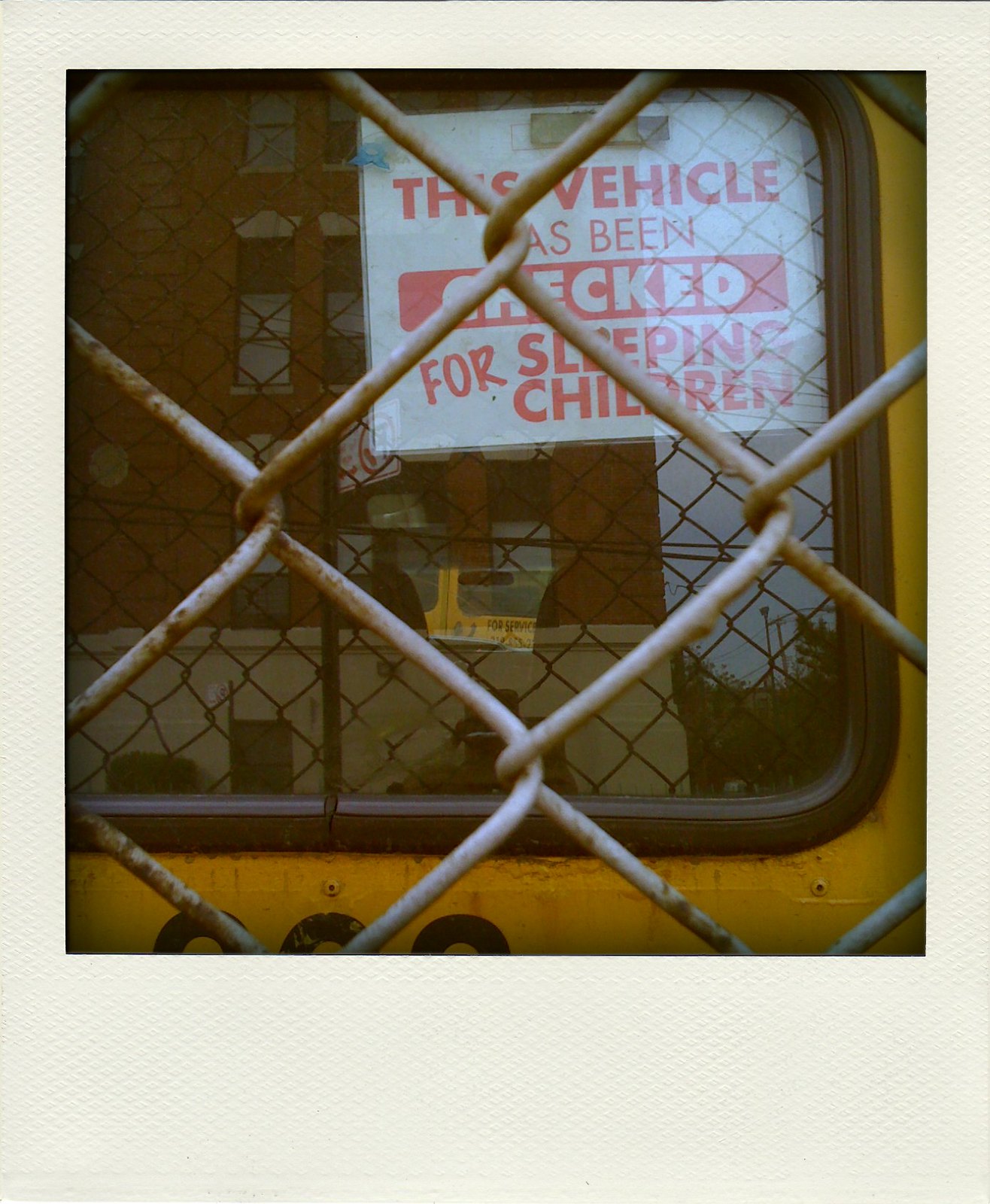In this detailed photograph, the viewer's focus is drawn to a white, rust-speckled, chain-link fence occupying the foreground. The fence spans about two to three squares in both the vertical and horizontal dimensions, suggesting a close-up shot. Through the weathered fence, a portion of a yellow school bus is visible. This includes the bus window, bordered in black rubber, which occupies the upper right portion of the visible area. The window features a white poster with red lettering stating, "This vehicle has been checked for sleeping children." Reflecting in the bus window is a detailed scene consisting of a multi-story brick building with numerous windows, green shrubbery, and a structure with a rust-colored brick facade atop a yellow base, behind the camera's perspective. The entire photograph is framed with a light gray border, further emphasizing the close-up focus on the interaction between the metal fence and the bus.